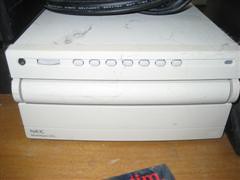The image depicts a compact, vintage-looking white device resembling an external CD-ROM drive. The unit stands approximately three inches tall, six inches wide, and six inches deep, with a design suggesting it might be an add-on for a computer tower, though it's self-contained. On the top portion of the device, several buttons are visible, while the front houses a central slot or drawer, likely a CD tray that opens with a push button. 

Notable features include scuff marks or stains on the surface, black text in the bottom left corner, and a thick black cable positioned towards the back, with white writing on the cable itself. The device rests on a light brown table, identifiable by a scratch mark at the front. Nearby, there is a piece of grayish paper with red letters on the edge.